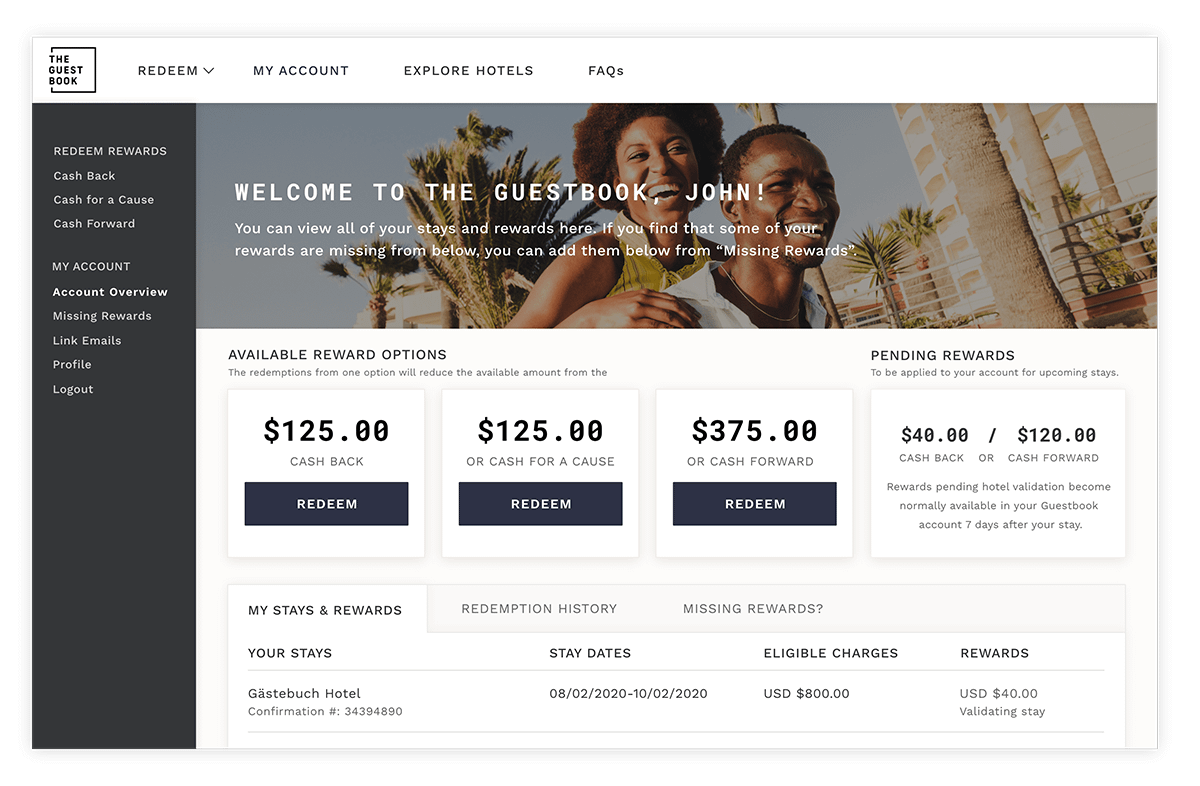This is a detailed screenshot from the Guestbook website. The white header at the top includes the Guestbook logo on the left, followed by navigation categories: Redeem (with a drop-down icon), My Account, Explore Hotels, and Facts. Below the header, the left side of the page features a vertical blue column with two main sections. The first section is "Redeem Rewards," which expands to show subcategories: Cash Back, Cash for a Cause, and Cash Forward. The second section is "My Account," comprising five subcategories: Account Overview, Missing Rewards, Link Emails, Profile, and Logout. The "Account Overview" subcategory is currently selected.

To the right of this vertical menu is the Account Overview page. The top of this section is dominated by a large photographic background depicting a happy couple, with the woman riding on the man's back. Overlaid on the left side of this image is a friendly welcome message: "Welcome to the Guestbook, John. You can view all of your stays and rewards here. If you find that some of your rewards are missing from below, you can add them from Missing Rewards." Below this message, a detailed breakdown of John's earned rewards is displayed.